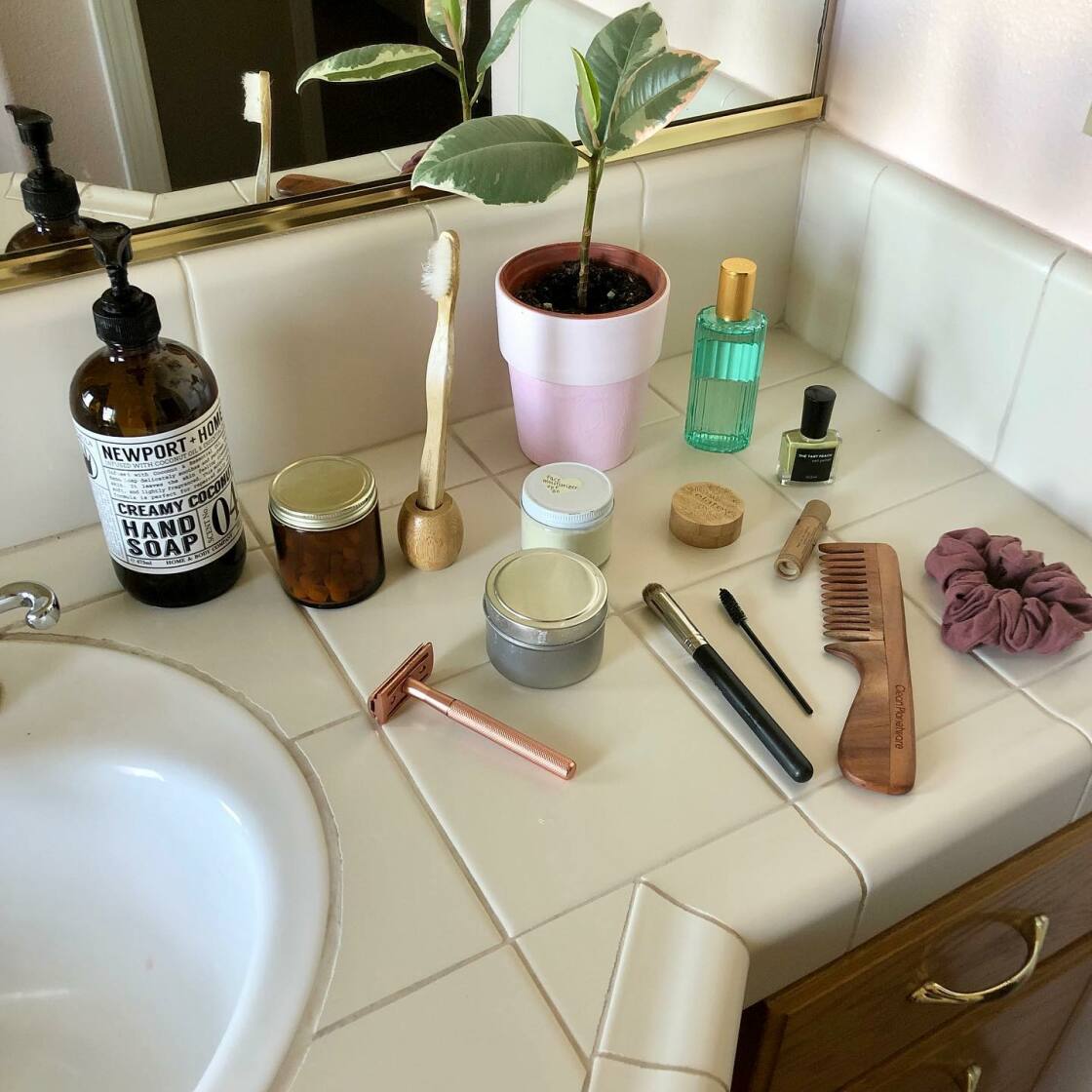This photograph, taken in an indoor bathroom setting, captures a detailed view of a countertop made of white square tiles with visible grout lines. In the bottom left-hand corner of the image, a flush-mounted white oval sink with a metal silver faucet is seen. To the right of the sink sits a dark bottle of Newton HOW Creamy Coconut Hand Soap with a pump. Adjacent to this is a closed jar containing a brown liquid and some brown beans. Next, a bamboo toothbrush rests in a matching bamboo holder. Further right, a pink pot holds a growing four-leaf plant, and in front of this pot stand two cylindrical jars—one white and one silver. Positioned in front of the silver jar is a metal reusable razor. To the right of this jar lies a makeup brush, followed by an eyelash brush, a brown plastic comb (bearing unreadable text), and a purple scrunchie. Nearby is a green bottle, likely aftershave, with a black cap. Above these items, a coaster can be seen, and in the background, the countertop is reflected in a gold-bordered mirror against a pink wall. Below the countertop, wooden cabinets with gold-colored handles are visible, completing this richly detailed snapshot of a bathroom's countertop.